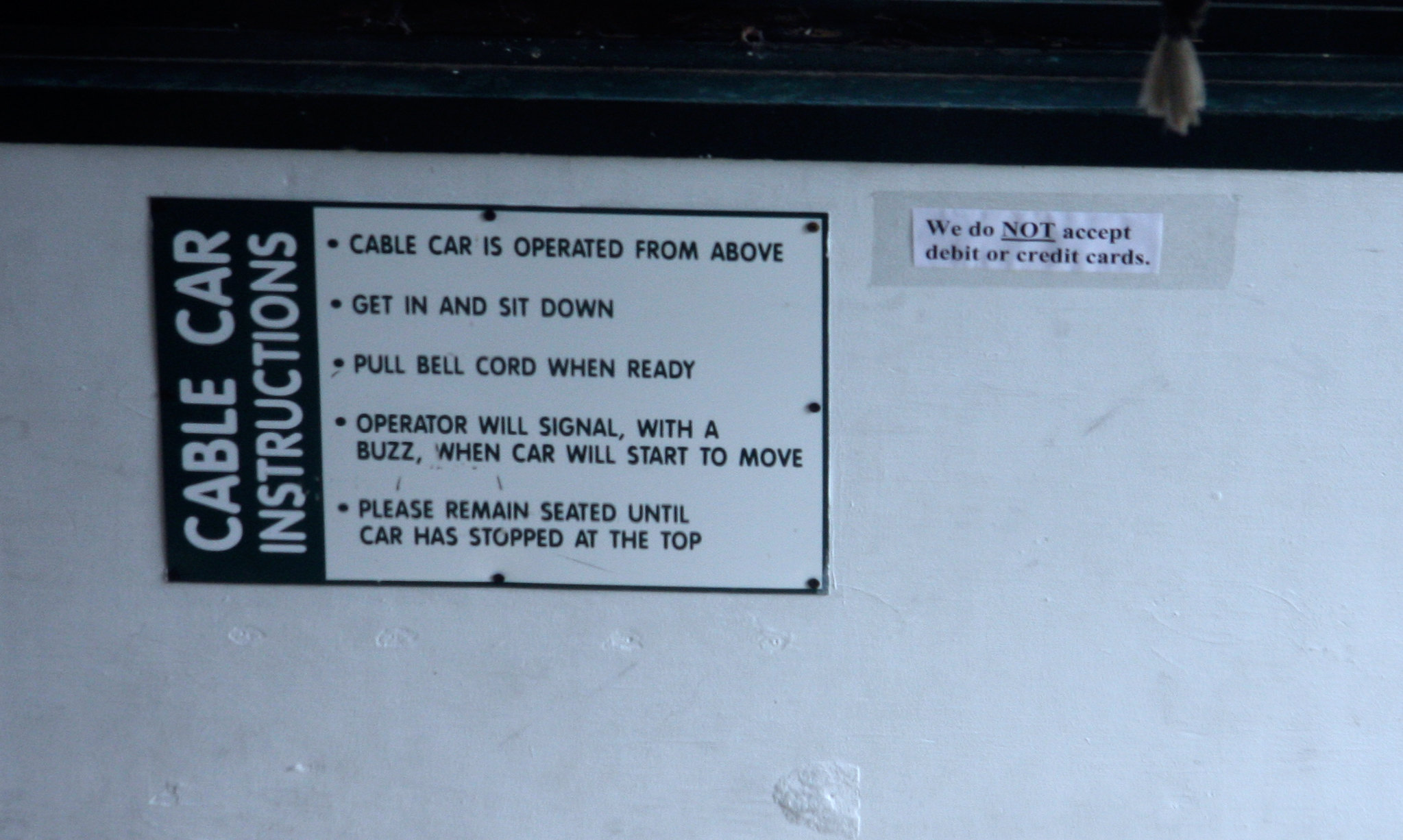The image captures detailed instructions for a cable car, prominently displayed on a white background with green and white coloring. The placard reads "Cable Car Instructions" with clearly listed steps: "Cable car is operated from above. Get in and sit down. Pull bell cord when ready. Operator will signal with a buzz when car will start to move. Please remain seated until car has stopped at the top." Additionally, a small paper card taped to the right of the main instructions states, "We do not accept credit or debit cards," indicating that cash is required for the ride. These instructions appear to be affixed to the side of the vehicle, ensuring that prospective riders are well-informed about the procedures and payment methods before boarding.